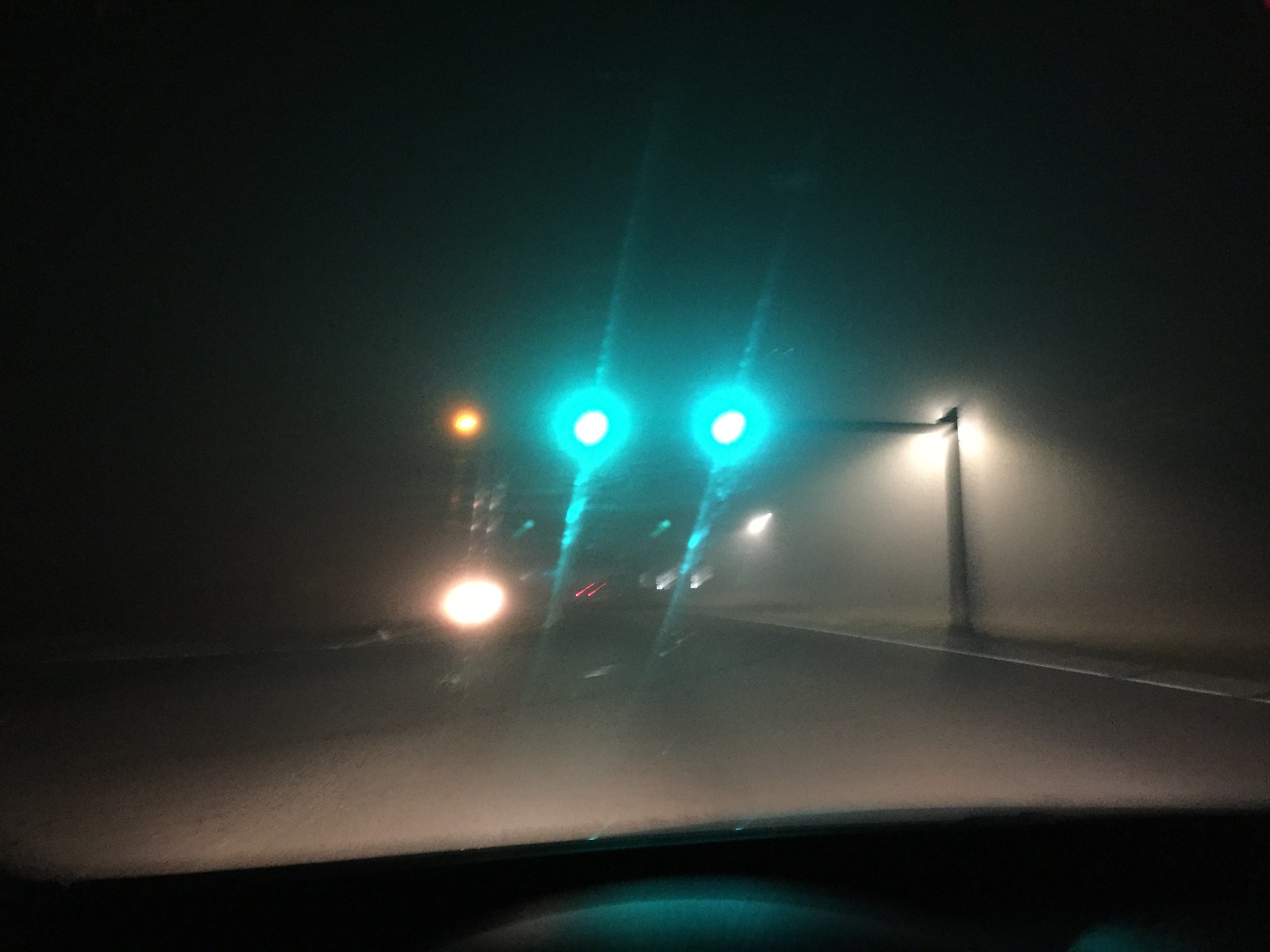This photograph captures a dark, night-time street scene viewed from inside a stationary vehicle, with the upper part of the dashboard and steering wheel in the foreground. The image is somewhat out of focus, adding a sense of distortion and blur to the lights. Through the windshield, two green traffic signals are visible, each attached to an L-shaped support pillar. Both green lights are surrounded by halos and rays of light extending up and down. The street ahead is dimly lit, with white, circular, glowing headlights from an oncoming vehicle approaching. The road appears mostly deserted. A high wall runs along the right side of the street, while in the distance, a tall building with a light on top, possibly orange, looms in the background. The dark sky envelops the entire scene, contributing to the overall obscured and surreal atmosphere.